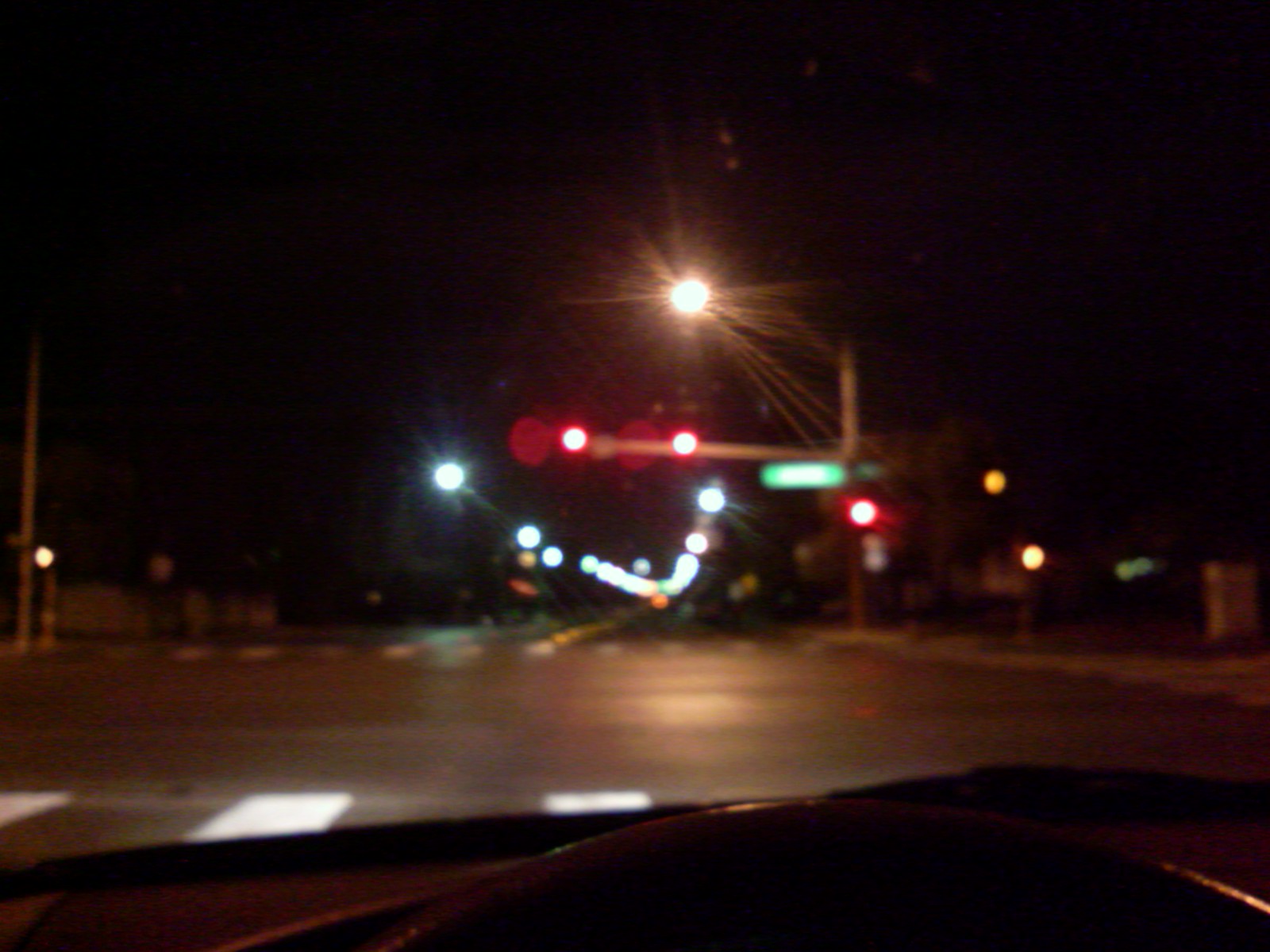This photograph, although blurry and out of focus, captures a nighttime city scene from the perspective of someone inside a car. The sky is pitch black, highlighting a bright, round white light situated centrally in the image. Just below this light, there is a traffic signal pole adorned with three lit red lights and a green street name sign, the text of which remains unreadable. The photograph depicts a four-way intersection, with a long, straight road extending ahead, lined with numerous streetlights on both sides. Only a small section of the crossroad is visible in front of the car, delineated by a painted crosswalk.